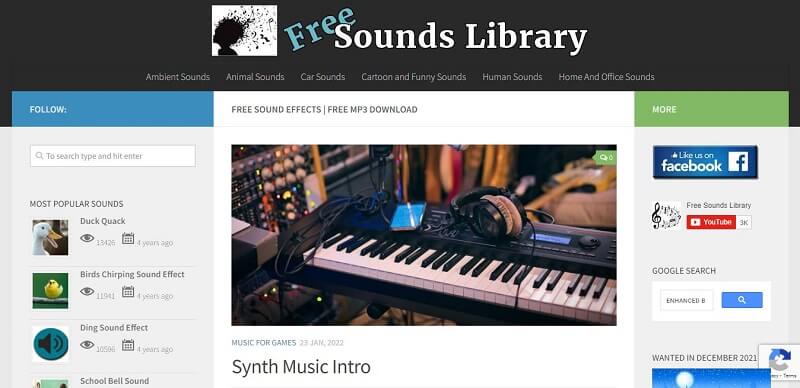The image showcases a website dedicated to providing free sound effects. The site features a gray border at the top and prominently displays a white square with a striking black silhouette of a person facing left, their hair blown upwards with musical notes emerging from it. To the right of this graphic, the text "Free Sounds Library" appears, with "Free" angled diagonally in blue, and "Sounds Library" in white.

Beneath this header, a gray font lists various categories: Ambient Sounds, Animal Sounds, Car Sounds, Cartoon and Funny Sounds, Human Sounds, and Home and Office Sounds. On the left side, a blue banner labeled "Follow" invites interaction. Below it, a search bar prompts users to "To Search, Type, and Hit Enter."

The "Most Popular Sounds" section highlights some top picks: Duck Quack, Bird's Chirping Sound Effect, Ding Sound Effect, and School Bell Sound. To the right, within a white background area, there are further offerings: Free Sound Effects, Free MP3 Download, Synth Music, and Intro Music for Games. An accompanying image shows a keyboard, headphones, and a cell phone.

The site also encourages social media interaction with prompts to "Like Us on Facebook" and "Free Sounds Library on YouTube." Additionally, at the bottom right, a search field enhanced by Google, denoted with a blue search icon and the letter "B," offers further navigation capabilities.